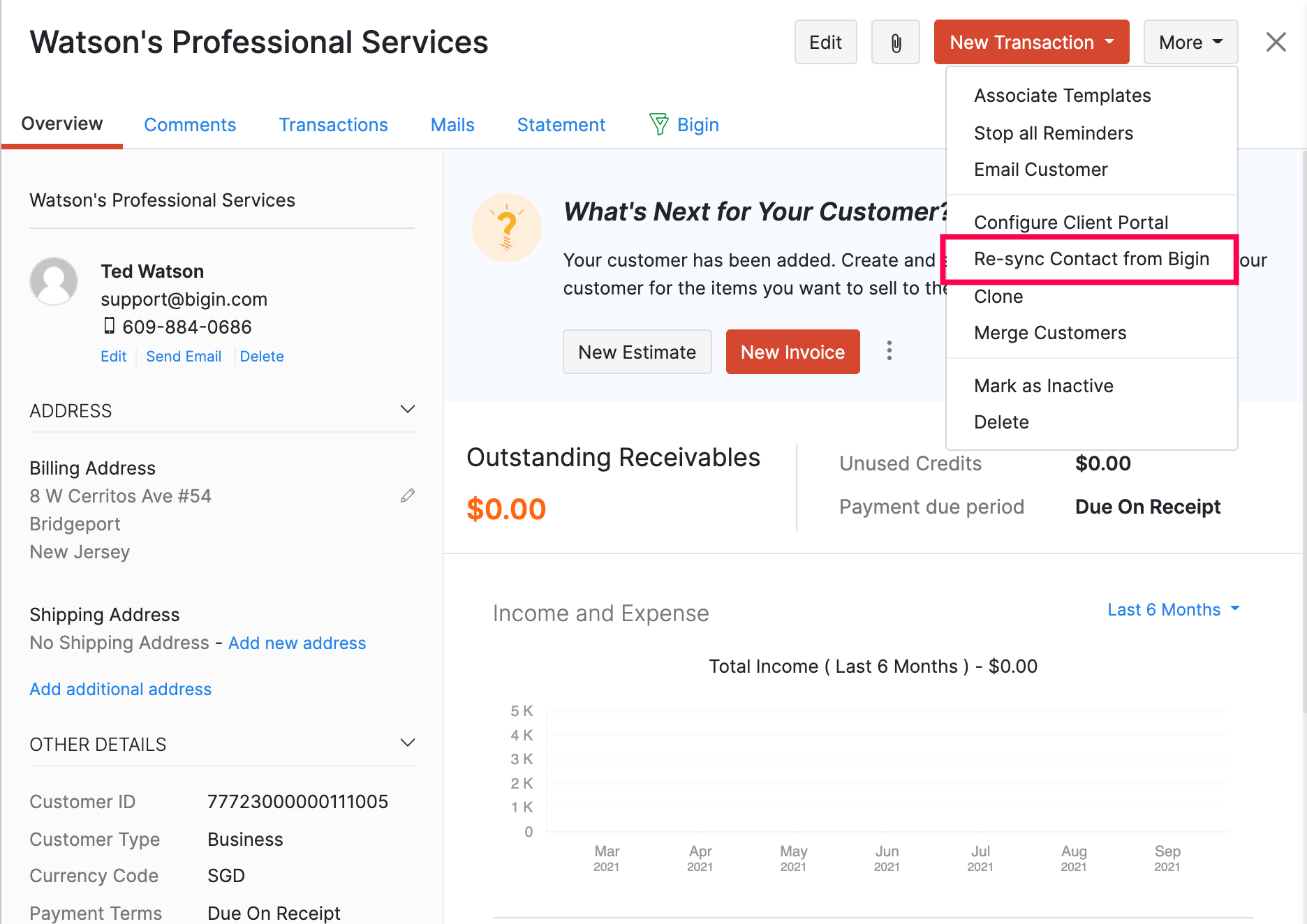**Caption:**

The image displays the backend dashboard of Watson Professional Services on what appears to be a Google Business platform. The dashboard is designed for business owners, providing various tabs and sections such as Overview, Comments, Transactions, and Mail Statements. "Overview" is highlighted, indicating it is the active section.

Key details about the business are prominently displayed, including the main contact, Ted Watson, whose email is ted.watson_support@login.com or ted.watson_support@bigin.com, and who can be reached at 609-884-080686. The dashboard also shows the billing address and other business-related information.

The most notable feature in the image is a section under "New Transactions" where the fifth box is circled in red. This box is titled "Resync Contact from Bigin" and is highlighted, suggesting a particular importance or a need for action. Additionally, the dashboard contains other sections that include details on outstanding receivables and the shipping address, providing a comprehensive view of the business operations.